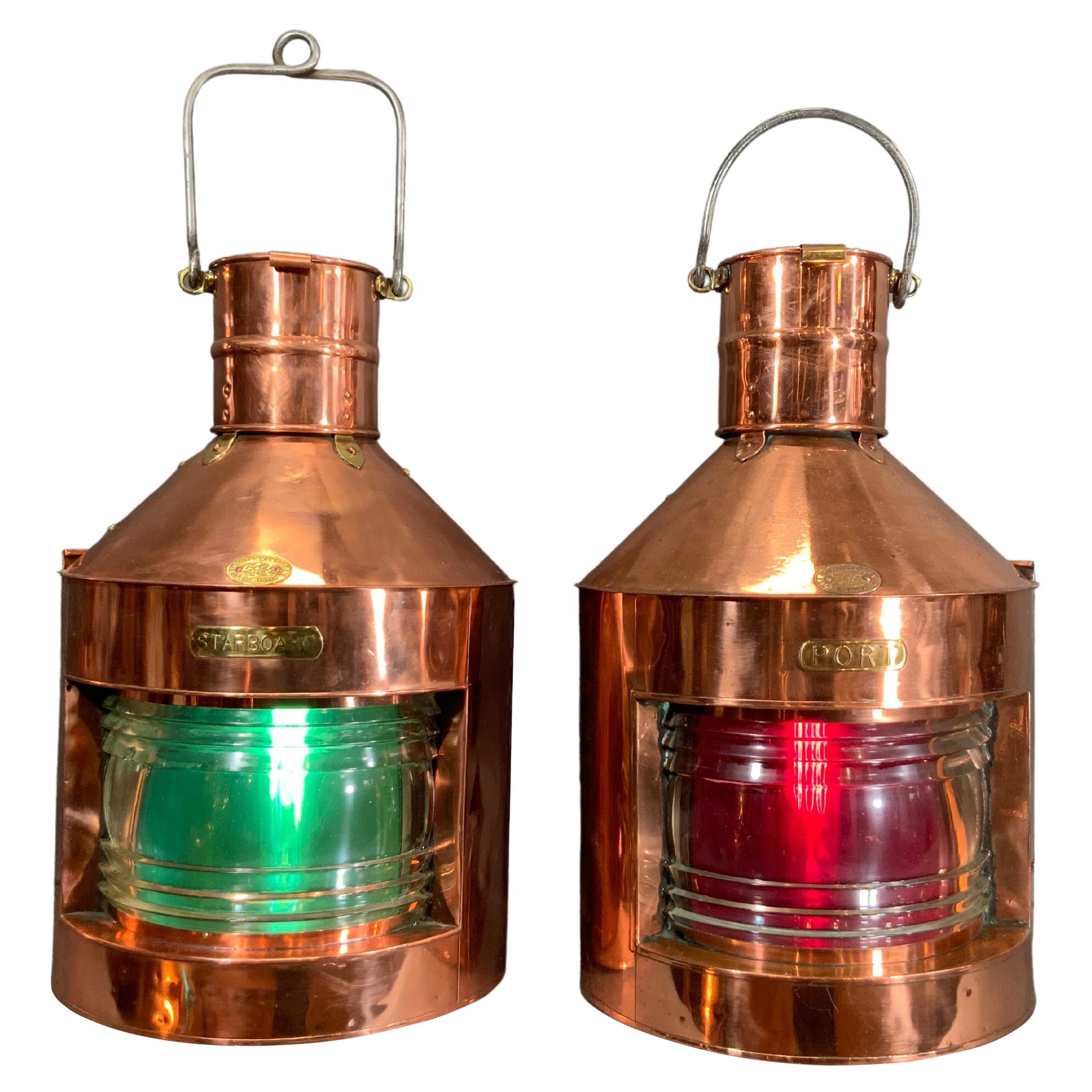The image shows two shiny brass lanterns, each meticulously designed for nautical purposes. These cylindrical lanterns feature inverted funnel-shaped tops with hooks for hanging; the Starboard lantern has a distinctive square-shaped hook, while the Port lantern has a semi-circular hook. Both lanterns have transparent chambers revealing colored glass lamps inside, indicating their functional use in maritime navigation. The Port lantern contains a red lamp, and the Starboard lantern contains a green lamp. Each lantern is clearly labeled, with "Starboard" inscribed on the green-lighted one and "Port" on the red-lighted one, which helps in identifying the left and right sides of a boat.